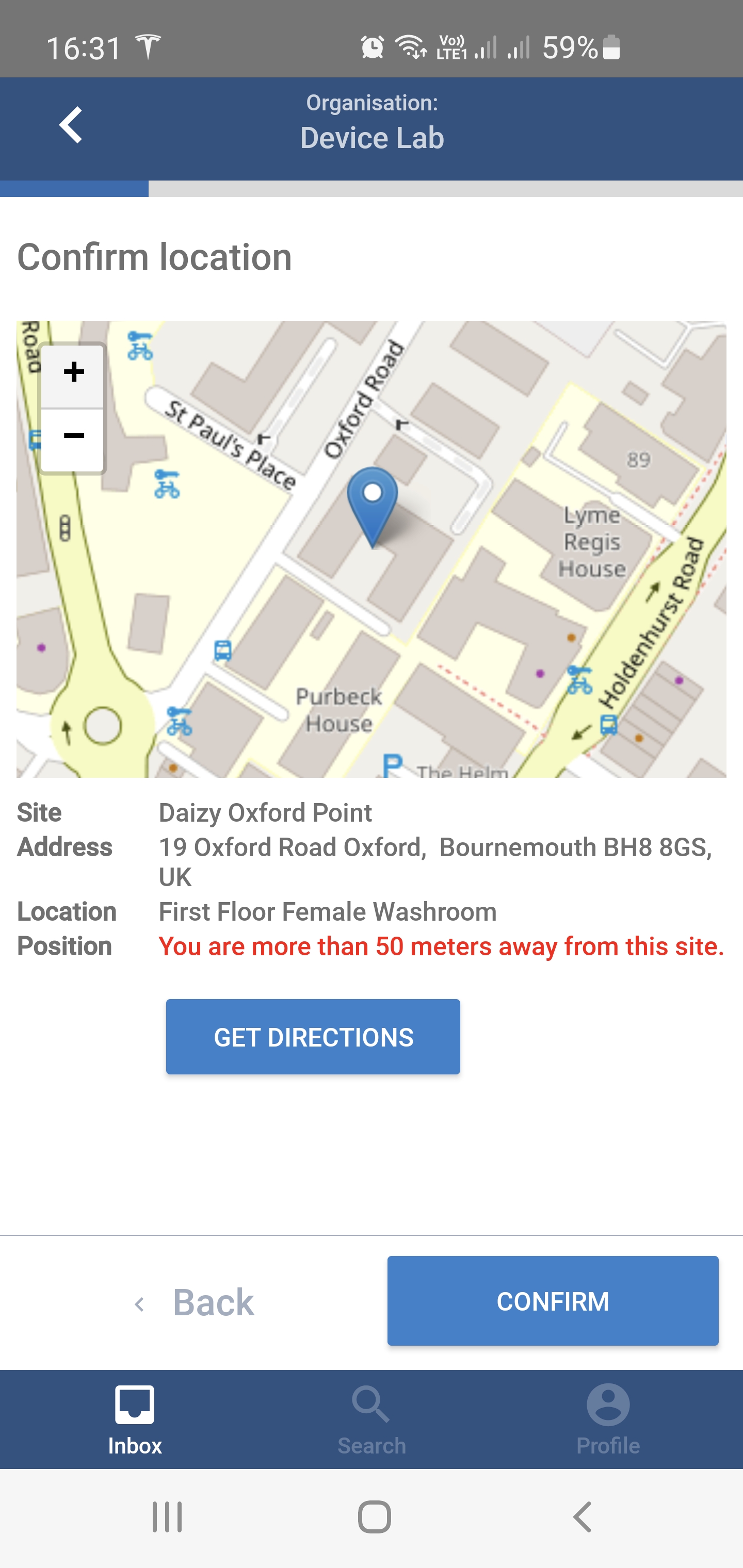The screenshot captures a smartphone displaying military time at 16:31 (4:31 PM) with a battery life of 59%. At the top, a blue banner indicates a navigation to "Device Lab" under the organization section. Below, a white bar prompts the user to "Confirm Location." The map displayed shows the location of the Device Lab between Hiddenhurst Road and Oxford Road. The identified site is named "Dazy" (spelled with a 'Z'), located at 19 Oxford Road, Oxford, Bournemouth, BH8 8GS, United Kingdom. The specific target location is the first-floor female washroom of this site. The user seems to be in search of something, as indicated by a note stating they are more than 50 meters away from the site. The interface provides options to either go back or confirm the location.